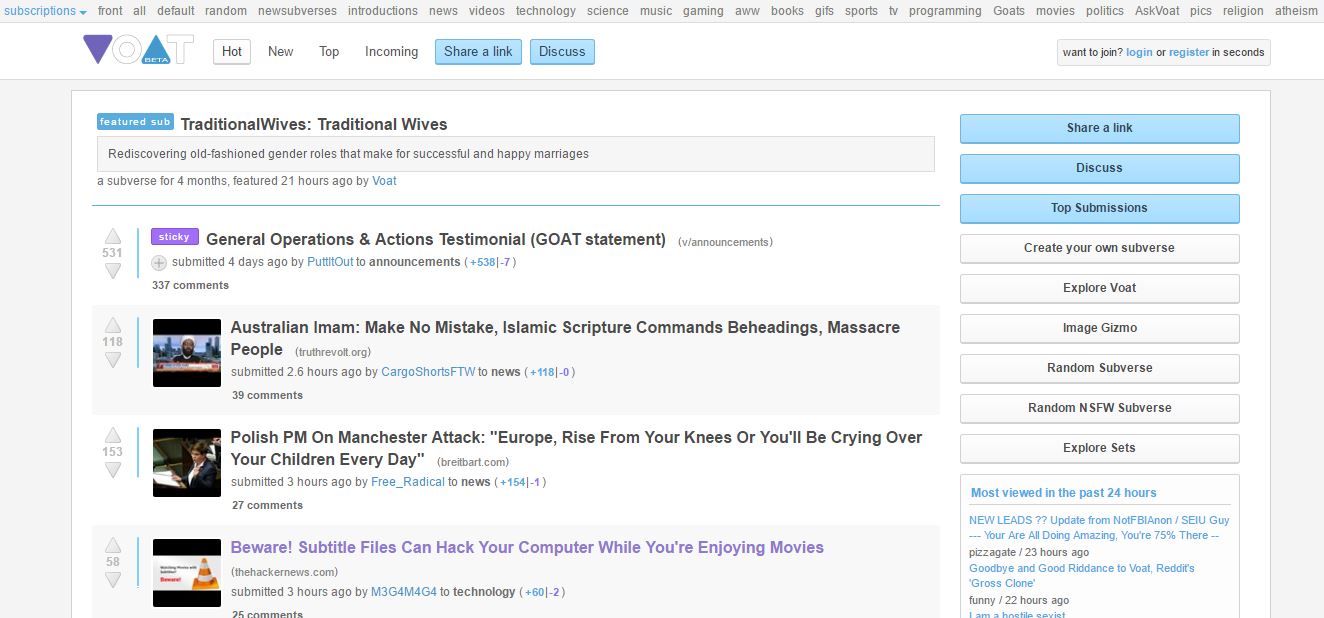This image features a highly detailed and varied page layout, separating content into distinct sections:

In the main section of the page, there's a segment about traditional wives rediscovering old-fashioned gender roles that purportedly lead to successful and happy marriages. Accompanying this information is a sticky note labeled "General Operations and Actions Testimonial (GOAT) Statement," which was submitted four days ago.

Below this content, on the left side, there is an image of a person appearing to speak on a television screen. The caption reads: "Australian Imam: Make no mistake, Islamic scripture commands beheadings, massacre people," submitted 2.6 hours ago, and it has garnered 39 comments.

Adjacent to this, another image displays a woman standing at what seems to be a podium, holding several pieces of paper. The caption reads: "Polish PM on Manchester attack: Europe, rise from your knees or you'll be crying over your children every day," submitted three hours ago.

The final image in this segment features an image with both top and bottom black borders, displaying blurry text and the bold word "BEWARE" next to an orange and white striped safety cone. It has a title "Beware" and a subtitle "Files can hack your computer while you're enjoying movies."

On the right side of the page, there's a column dedicated to community interaction. At the top, it says "Share a link" in blue. Below this are subsequent blue boxes labeled "Discuss" and "Top submissions," followed by additional colored rectangles with prompts like "Create your own subverse" and "Image gizmo."